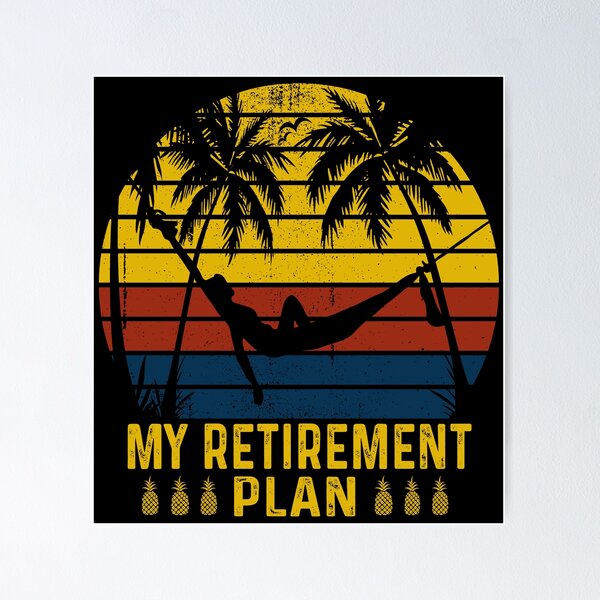The image portrays a poster against a black background centered around the text "My Retirement Plan" in bright yellow at the bottom. Flanking the word "plan" are three pineapples on each side. Above the text, a circular illustration depicts a person leisurely lying in a hammock. The circle is divided into three horizontal sections: the top third is yellow, the middle third is red, and the bottom third is blue. At the top of the yellow section, two birds are situated amidst two palm trees on either side. The person in the hammock is shown with one leg bent and arms hanging down, giving a relaxed vibe. Overall, the composition has an abstract artistic style reminiscent of decorative prints one might find in beachside gift shops.